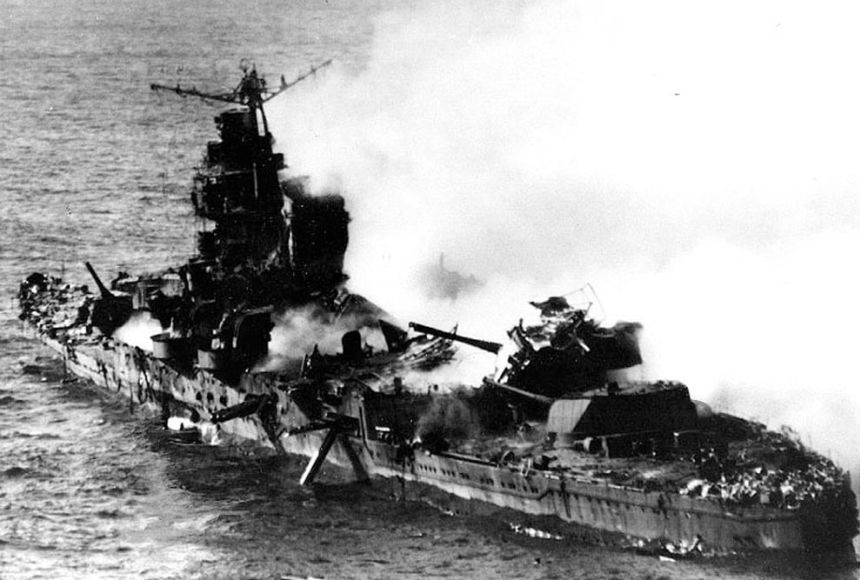In this evocative black-and-white photograph, a World War II battleship is captured in a state of severe disrepair and apparent demolition. Listing heavily to the right, the ship appears as though it might sink, with sections that are clearly corroded and other parts that seem to have broken off or been bombed multiple times. The vessel is adorned with several gun turrets, including one prominently positioned at the bow; however, some gun barrels are pointed into the water, indicating components have likely fallen off. A thick plume of smoke emanates from the ship, particularly from the front turret, enveloping the right side of the image and obscuring the water beneath it. The overall scene is one of high contrast, emphasizing the stark, dark hues of the battered ship against the surrounding sea, which shows some gentle waves, though the water itself is not particularly turbulent. The dramatic angle and intense atmosphere of this image evoke the chaos and destruction of wartime, with smoke consuming the upper right quadrant and parts of the ship nearly indistinguishable through the haze.